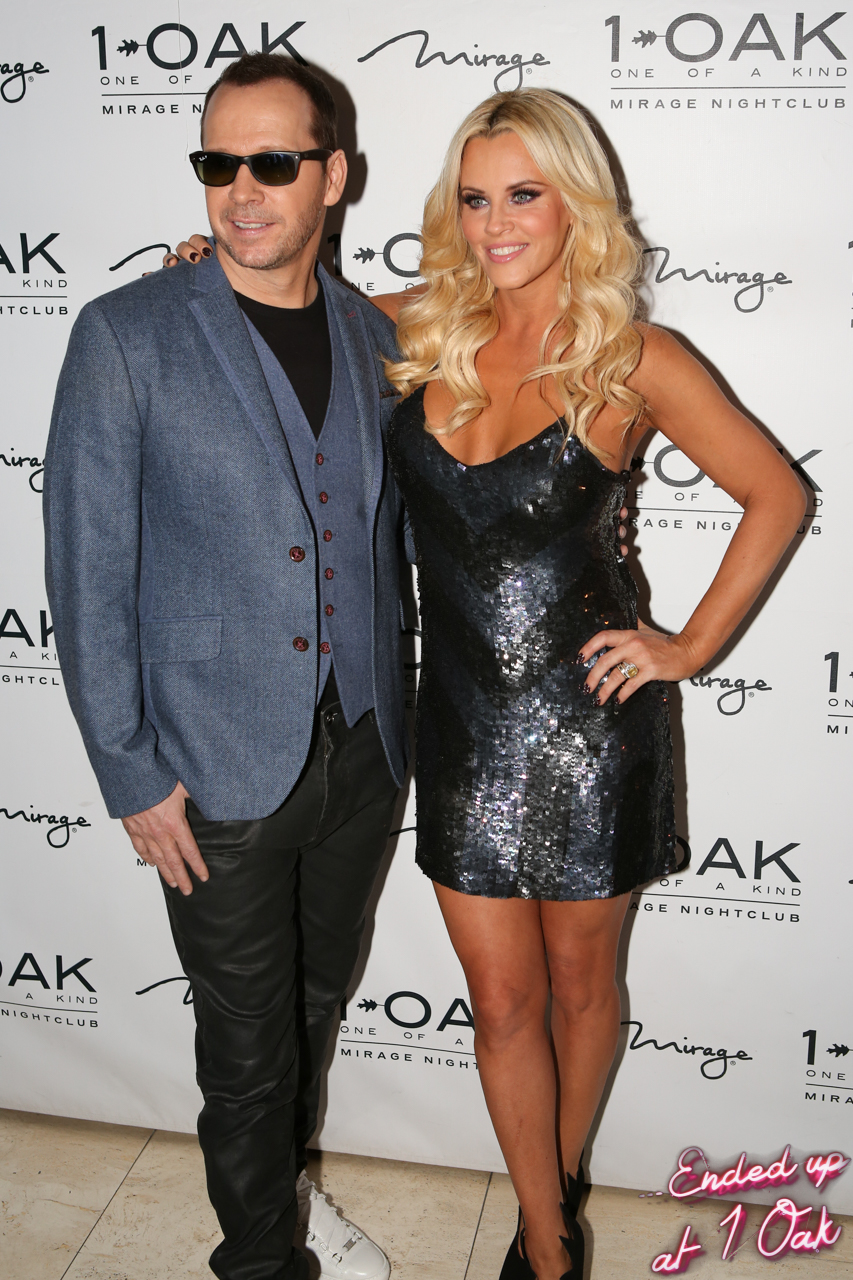This photograph captures a young couple, likely in their early to mid-twenties, standing in front of a white step-and-repeat banner adorned with sponsorship logos including, "One Oak Mirage," "One Oak," and "One of a Kind Mirage Nightclub," all in black text. The woman, who has shoulder-length blonde hair styled in slight waves, is wearing a strapless black sequined mini dress along with black shoes. Her nails are painted black, and she is seen smiling with her teeth showing. A wedding ring is visible on her finger, and she is posed with her right leg crossed in front of the left while her right hand is draped around the man next to her. The man standing to her right sports short brown hair and dark sunglasses. He is dressed in dark leather pants or possibly black jeans, a navy blue jacket over a navy vest, and a black shirt underneath. The lower right corner of the image features a pink neon-colored watermark that reads, "Ended up at One Oak".